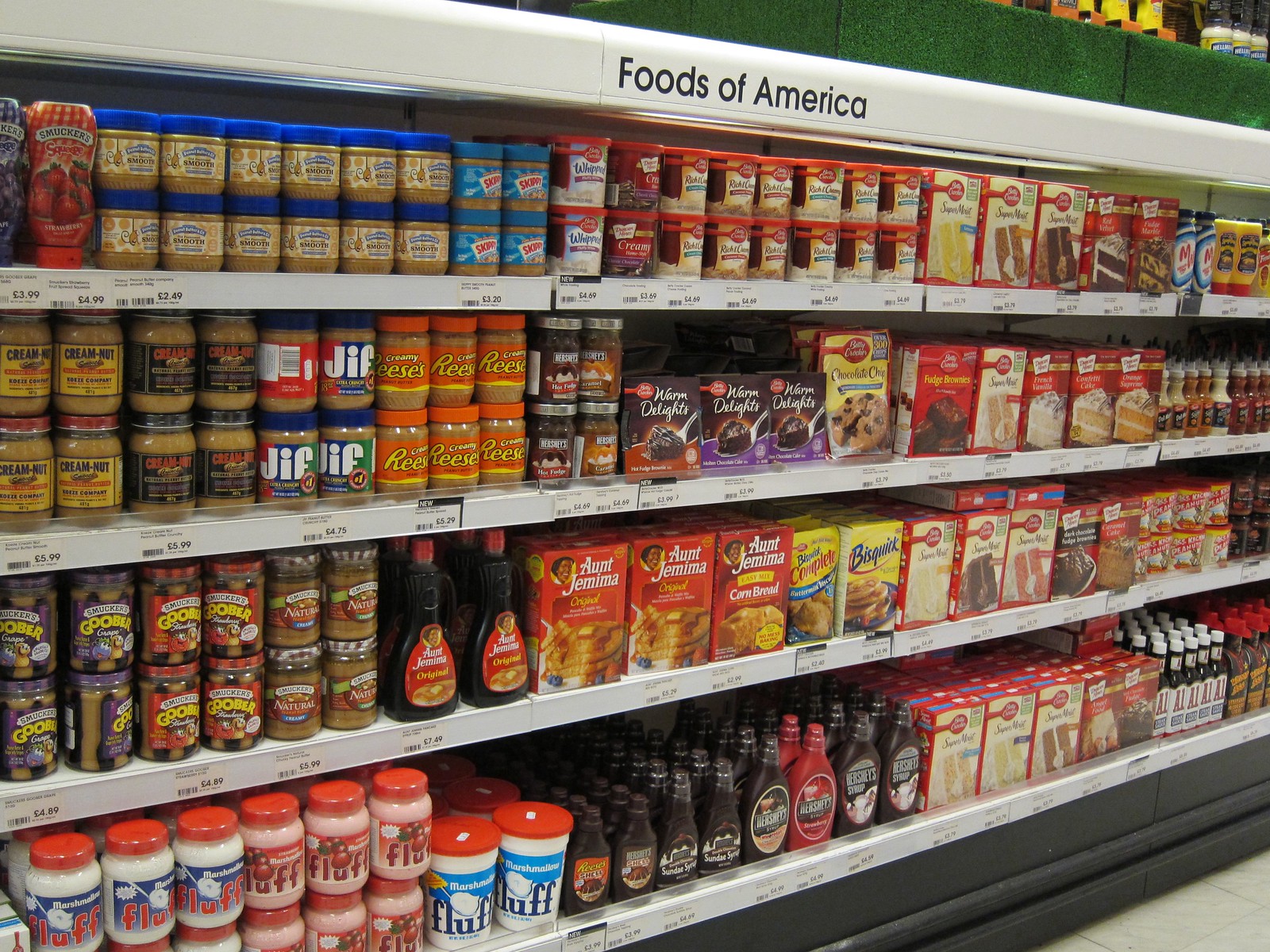This photograph captures a well-organized aisle in a grocery store, featuring pristine white metal shelves and polished white tile floors. Prominently labeled "Foods of America" at the top of the shelves, the display showcases a diverse array of American food products. Iconic brands such as Smucker's Jelly in grape and strawberry, Skippy Peanut Butter, Jif Peanut Butter, Reese's Peanut Butter in its distinctive orange jar, and Goober Peanut Butter are lined up on four shelves dedicated to various peanut butter varieties. The shelves also feature Betty Crocker items, including Whipped Frosting, Rich and Creamy Frosting, Cake Mixes, and Warm Delights, as well as Duncan Hines Cake Mixes. You can also spot Miracle Whip Salad Dressing, Marshmallow Fluff in pink and white containers with red tops, Hershey's Chocolate Syrup, Bisquick Pancake Mix, and Aunt Jemima Cornbread Mix. In addition to these popular items, various sauces such as mayonnaise and A1 sauce are on display. Each product has a clearly marked price, ranging from $2.49 to $5.99, emphasizing the organized and consumer-friendly presentation of the aisle.